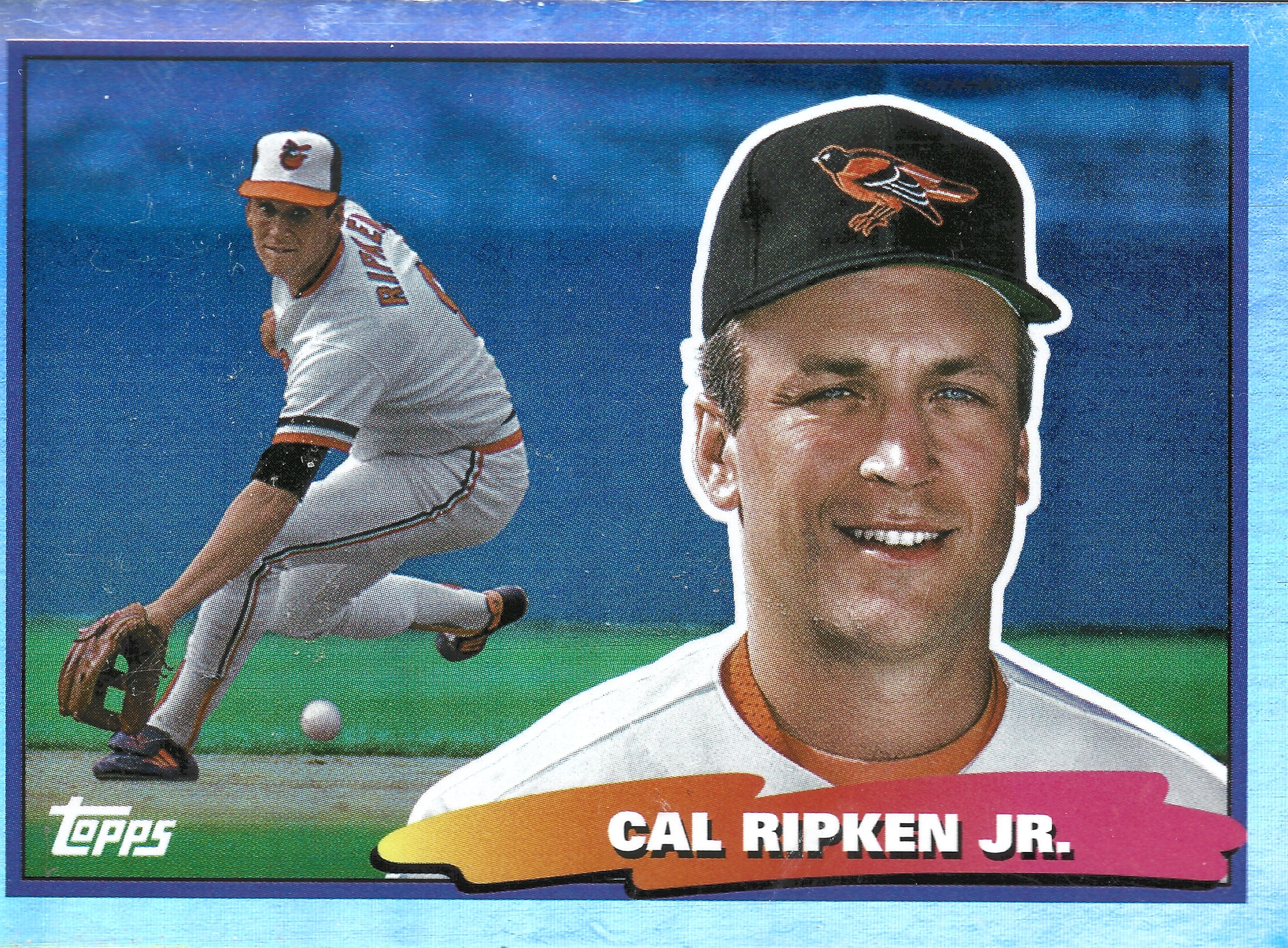This is a detailed color image of a vintage Topps baseball card featuring Cal Ripken Jr. On the left side of the card, there is an action shot of Cal Ripken Jr. fielding a ground ball on the infield, with a green grass background and a blue outfield wall behind him. He is depicted wearing his Baltimore Orioles uniform with a white jersey, orange under-jersey, and a white hat with an orange brim. On the right side, there is a photoshopped cutout of his head and shoulders in a close-up view, where he is shown wearing a black cap adorned with a bird patch, consistent with the Orioles hat. On the lower right corner of the card, there is a yellow-orange and light pinkish tag displaying his name, "Cal Ripken Jr.," in white text. The iconic Topps logo, T-O-P-P-S, is prominently situated in the lower left corner, marking its authenticity as a classic baseball card.